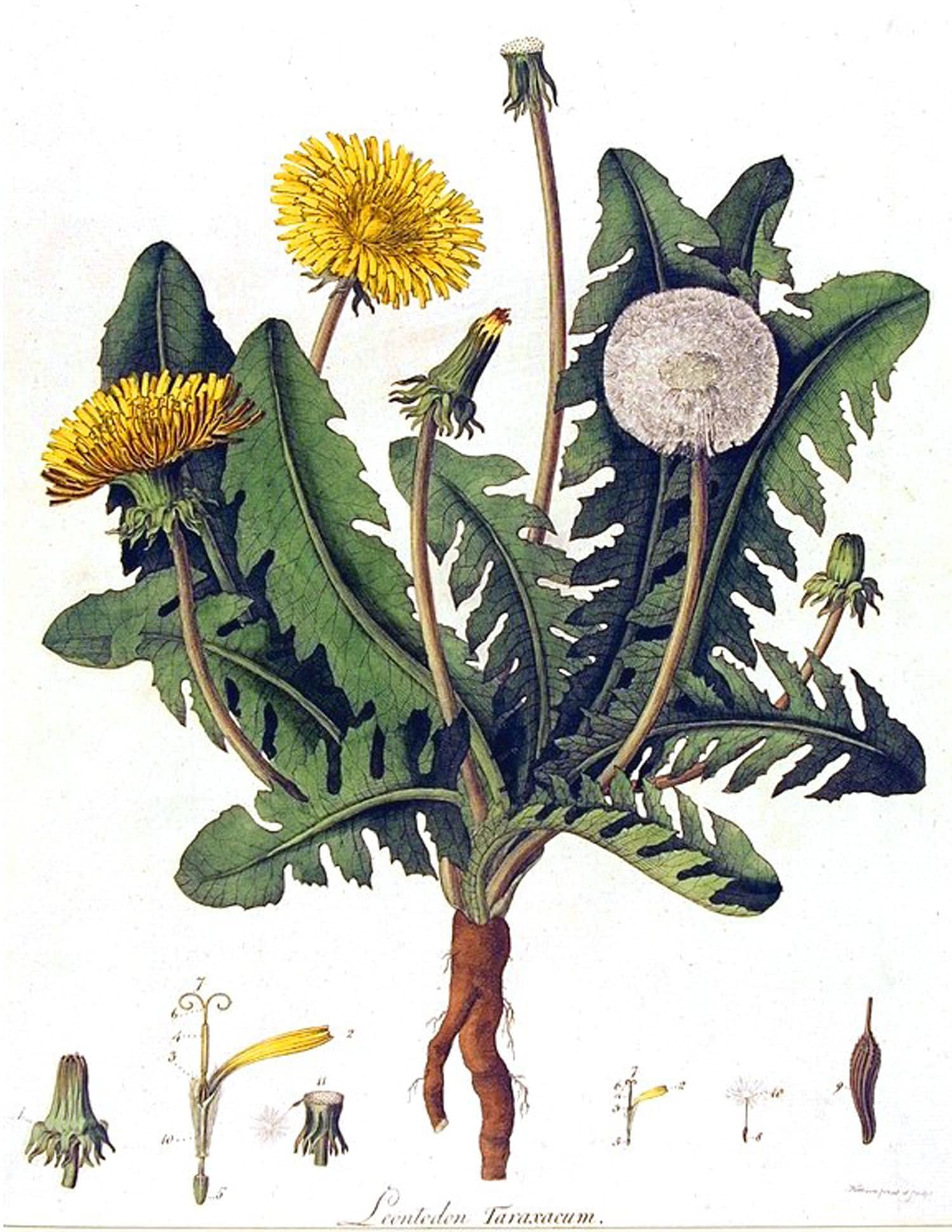This detailed illustration appears to be the work of an artist, meticulously rendered on paper. Dominating the center of the composition, a brown root resembling the texture of a sweet potato, extends upwards from the ground. Emerging from this root are long, green leaves and several intricate flowers. Among these, there are two vibrant yellow blossoms and one mature, white, puffy dandelion-like flower with delicate seeds ready to be dispersed by the wind. Additionally, several flower buds are still waiting to bloom. 

At the bottom center of the image is the text "Lentatum Taraxacum," suggesting a botanical theme. On the bottom right, finer text is inscribed, although it is too small to be legible. Further along the bottom edge, a series of smaller, detailed floral illustrations are present, each marked with numbers. However, no corresponding chart or legend is provided to elucidate these numerical labels. The overall scene is rich with botanical details, blending vibrant natural elements with an annotated scientific approach.